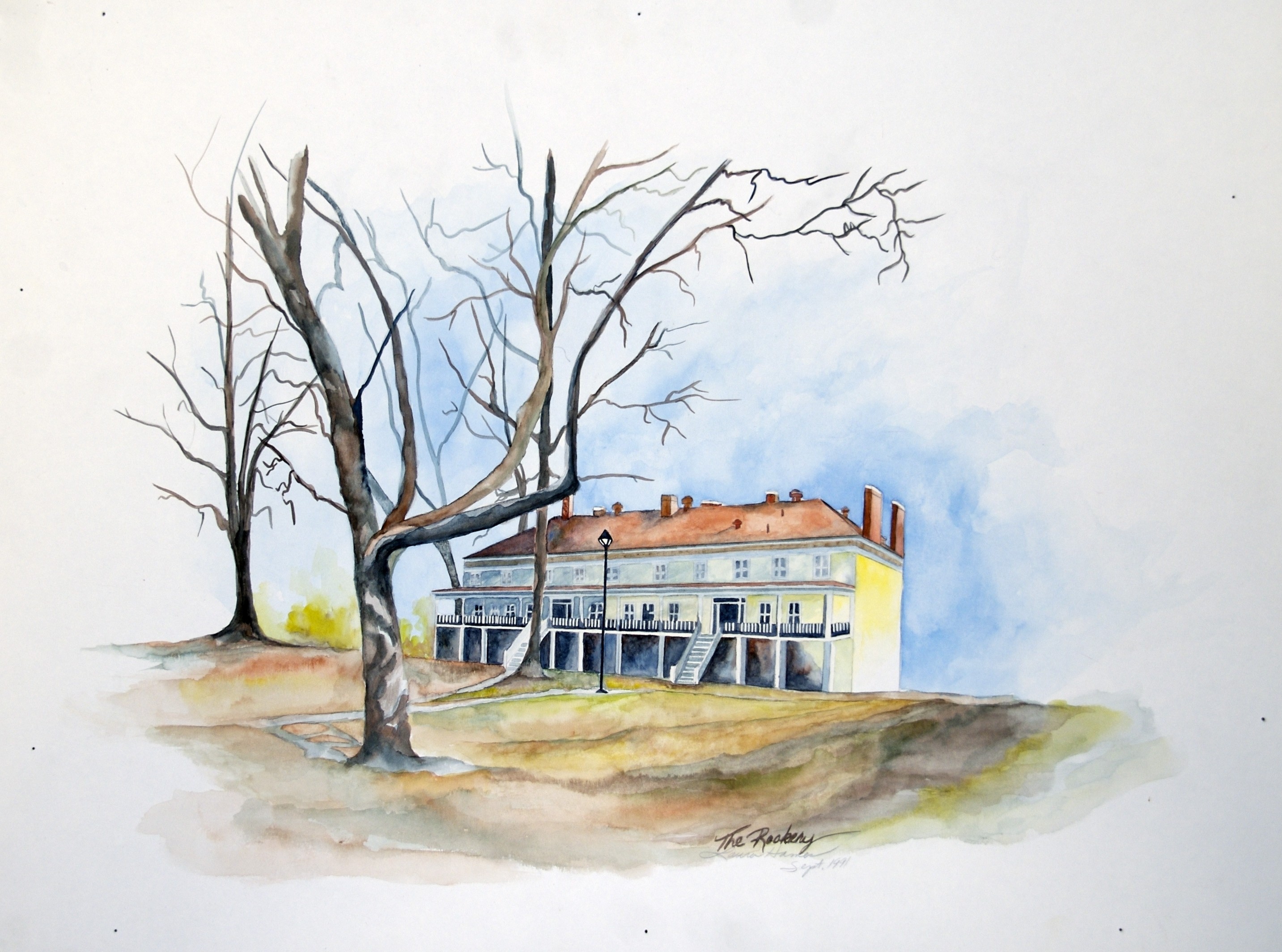This detailed painting is executed primarily in watercolor with pencil line drawings, and it depicts a stark winter scene centered around a colonial-style building. The building appears to be a long, narrow three-story structure with a white facade and a light red-brown sloped roof accented by several chimneys. Balconies adorn the building, supported by white columns, and twin staircases lead up to the second level from ground level. The building, possibly a hotel, stands on a hill, with a ground painted in shades of light brown to greenish tones. In the left foreground, two leafless trees stretch upwards, their dark brown branches possibly sprinkled with patches of snow. A black street lamp with a white lamp head stands nearby. The sky is painted blue with scattered white and gray clouds, and an intense fog or light gray haze envelops the scene, particularly around the edges, adding a sense of depth and mystery. The painting is signed in brown cursive at the bottom right, though the signature is partially illegible. The dimensions of the painting are approximately five to six inches in width and four to five inches in height, making it a small yet intricate depiction of a serene, wintry landscape.